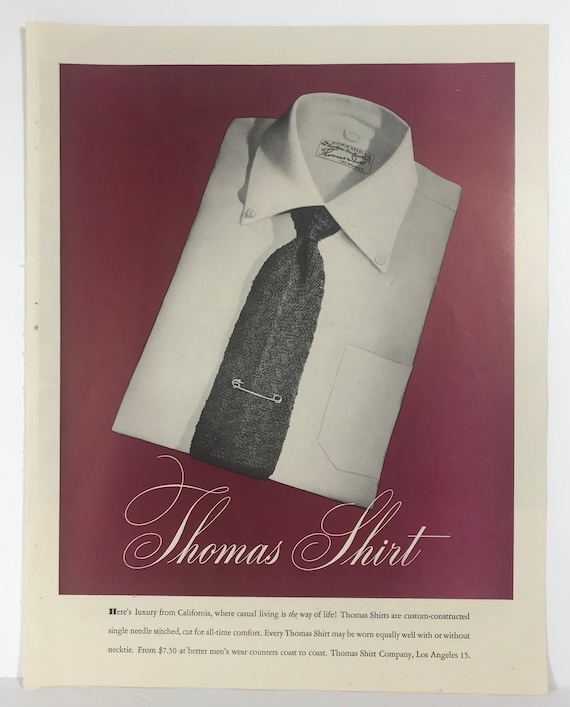This is a vintage advertisement for a white button-down business shirt, presented on a cream-colored, rectangular piece of paper in portrait orientation. The advertisement features a striking red (burgundy) rectangular background that occupies the top three-quarters of the image, showcasing a neatly folded white men's shirt with a button-down collar. The shirt is accessorized with a gray tie that appears to be made of a rough, possibly knitted or crocheted, material and secured with a safety pin. At the center of the image, the shirt is angled with the collar near the top right corner and the folded part facing the bottom left. Below the shirt, in elegant white script font, the text reads "Thomas Shirt." Further down, on a white background and in a black printed text, it states, "Here's luxury from California where casual living is the way of life. Thomas shirts are custom constructed single needle stitch cut for all time comfort." The advertisement is framed by a white matting that blends into what seems to be a white painted wall, resting on a gray tabletop or countertop. The overall depiction of the advertisement and its surrounding details exudes a sense of classic, luxurious style resonant with Californian casual living.